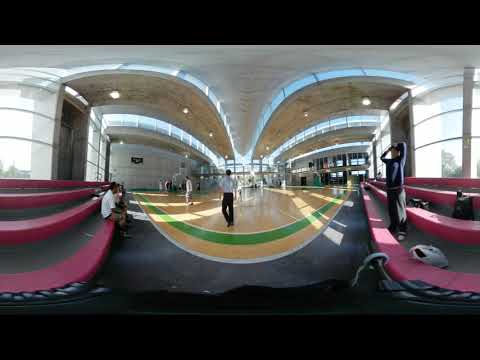The photograph showcases a vast, indoor area, likely part of a mall or large building. The floor is decorated with a striking combination of yellow, green, and gray, featuring a distinct green stripe. This is complemented by a reddish and black cushioned seating area that lines both sides of the wide hallway. The ceiling above is white, imbued with modern, abstract designs reminiscent of butterflies, and illuminated by embedded lights. The hallway culminates in visible doorways, suggesting entrances or exits. The presence of various people adds a dynamic aspect to the scene: individuals are seated on benches, standing on steps, and walking across the floor. One person is specifically noted in a navy blue sweatshirt and black sweatpants, standing with arms raised on the first step of the three concrete, red-painted steps. Another person wearing a black ball cap and white short-sleeved t-shirt is sitting on the steps, with a plastic shopping bag nearby. Large windows behind the steps allow natural light to pour in, enhancing the airy feel of this expansive and lively indoor space.